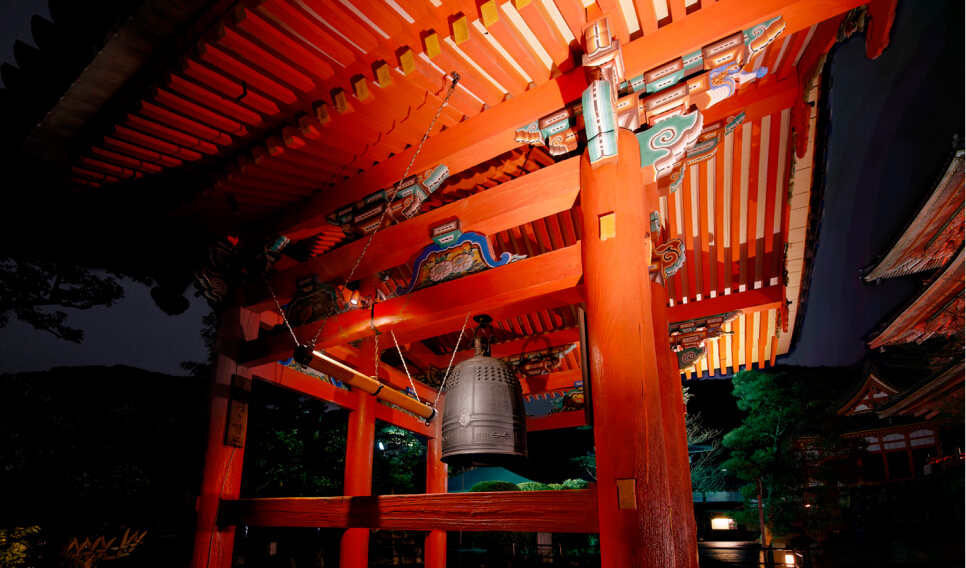The image depicts an orange pergola with round columns supporting a top structure made of orange wooden pieces. A dark gray metal bell hangs from the roof's center, reflecting a bit of light. At the junctions where the columns meet the roof, light teal patches intermixed with circular designs of teal, orange, and white can be seen. The background to the left and right is predominantly dark, suggesting nighttime, with a silhouette of trees to the left and some visible green trees on the bottom right. An orange square light and a smaller circular light are visible beneath the green trees. Rolling hills and the rooflines of pagodas are discernible in the distance. Some branches appear towards the upper left, partially obscuring a blue sky that peeks through the greenery.